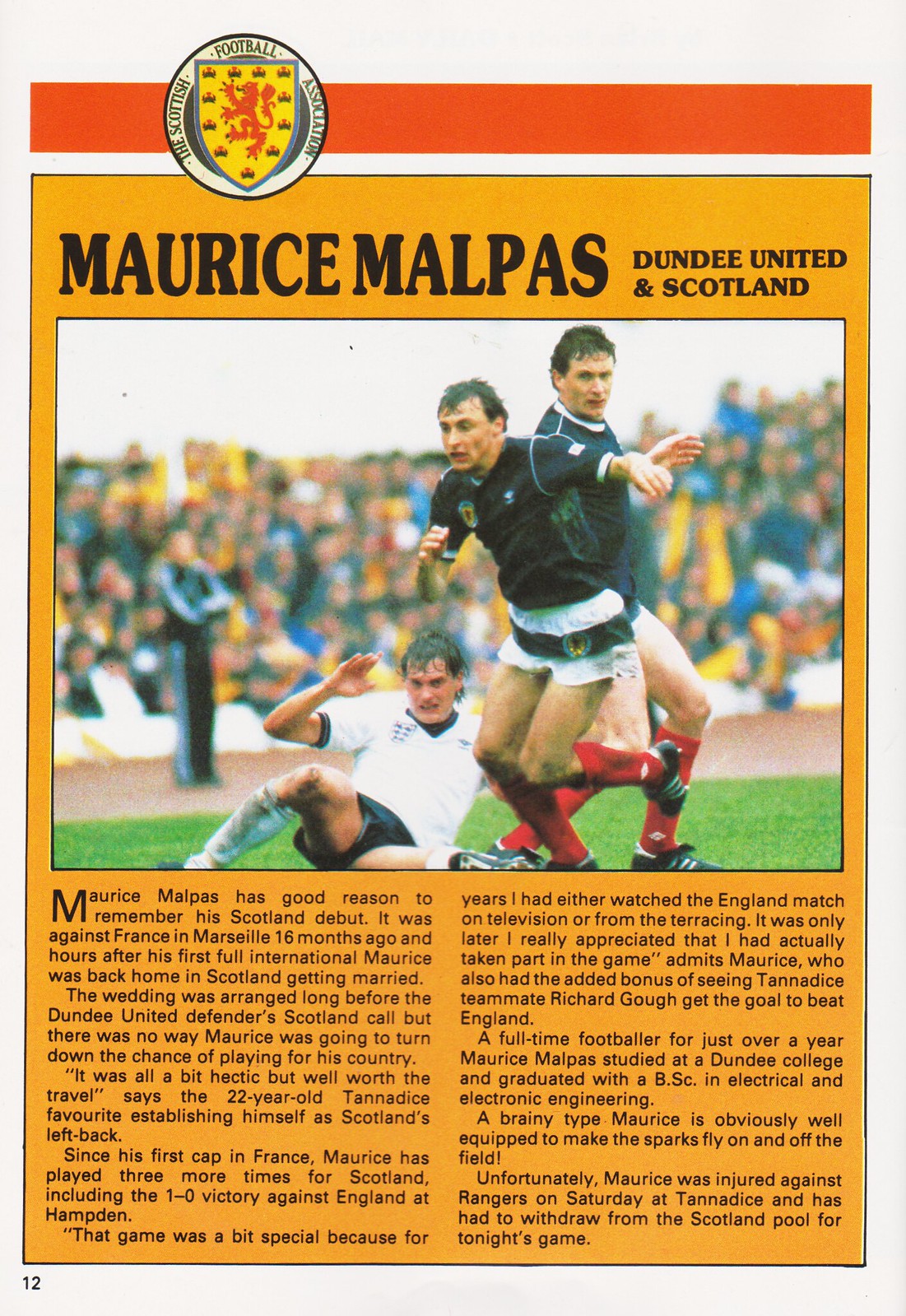The image features a vintage football program page set against a white background with a distinct orange theme. Dominating the top section is a darker orange horizontal stripe, overlaying which is an emblem situated near the upper left corner. The emblem reads "Scottish Football Association," encircling a shield adorned with an orange lion. Directly beneath this emblem, black text within an orange square lists "Maurice Malpas, Dundee United, Scotland." Prominently in the center of the page, a photograph captures the dynamic scene of three football players in action. One player dons an all-white uniform with black shorts, while the other two sport a black top, white shorts, and red socks, with a blurred crowd and grassy field in the background. Beneath this compelling image, two columns of black text narrate the context, including details of Maurice Malpas's notable Scotland debut against France in Marseille, culminating in his return to Scotland for his wedding. The page number "12" is indicated at the bottom, grounding this vibrant snapshot into a tangible piece of football history.